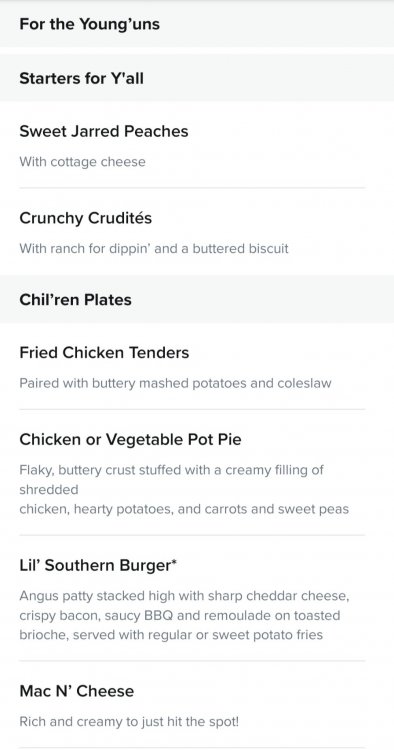**For the Youngins Menu**

Against an eggshell white background, the menu section titled "Ford Youngins" (stylized as "F-O-R-D Y-O-U-N-G-I-N-S") features a variety of options. The header text is in a lighter shade compared to the backdrop, making it subtly stand out. 

**Starters for Y'all (Y@A-L-L)**

- **Sweet Jared Peaches**
  - *With Cottage Cheese*

- **Crunchy Crudités (Crudités)**
  - *With Ranch for Dippin' and a Buttered Biscuit*

**Children Plates**

- **Fried Chicken Tenders**
  - *Paired with Buttery Mashed Potatoes and Coleslaw*

- **Chicken or Vegetable Pot Pie**
  - *Flaky Buttery Crust Stuffed with a Creamy Filling of Shredded Chicken, Hearty Potatoes, Carrots, and Sweet Peas*

- **Little Southern Burger (Burger®)**
  - *Angus Patty Stacked High with Sharp Cheddar Cheese, Crispy Bacon, Saucy BBQ Sauce, and Remoulade on Toasted Brioche, Served with Regular or Sweet Potato Fries*

- **Mac and Cheese (N)**
  - *Rich and Creamy to Just Hit the Spot!*